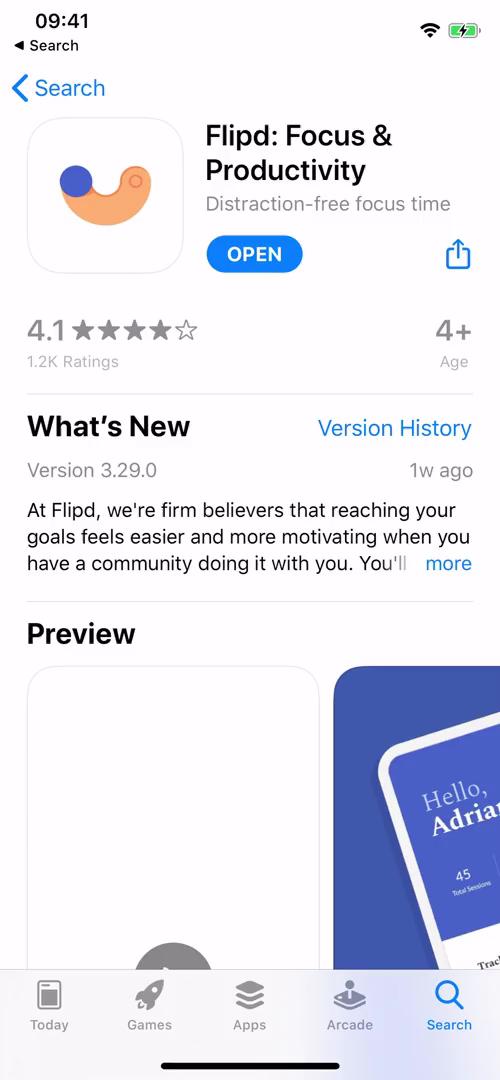The image showcases a detailed interface of a mobile app store on a light blue background at 09:41. It features a black search button at the top, followed by a blue search button with an arrow. Below, there is a white box with a blue outline containing a semi-circle with a blue circle on the left and a tiny red circle on the right. The text inside reads, "Flipped: Focus and Productivity, distraction-free focus time."

An open button in blue and a square with an up-arrow, also in blue, are present under the text. The app is rated for ages 4+ and has received 4.1 stars. Below this section, there is a small line separating it from further information, which includes a "What's New" section and "Version History" in blue text.

The details mention that version 3.29.0 was released one week ago. A snippet about the app reads, "At Flipped, we're firm believers that reaching your goals feels easier and more motivating when you have a community doing it with you."

Further down, there is a section titled "Yule" with "More" in blue text, followed by a preview that includes a purple square displaying "Hello Adrian" on a phone interface. There is a semi-circle in gray before reaching the bottom of the phone screen, which includes navigation options labeled "Today," "Games," "Apps," "Arcade," and "Search."